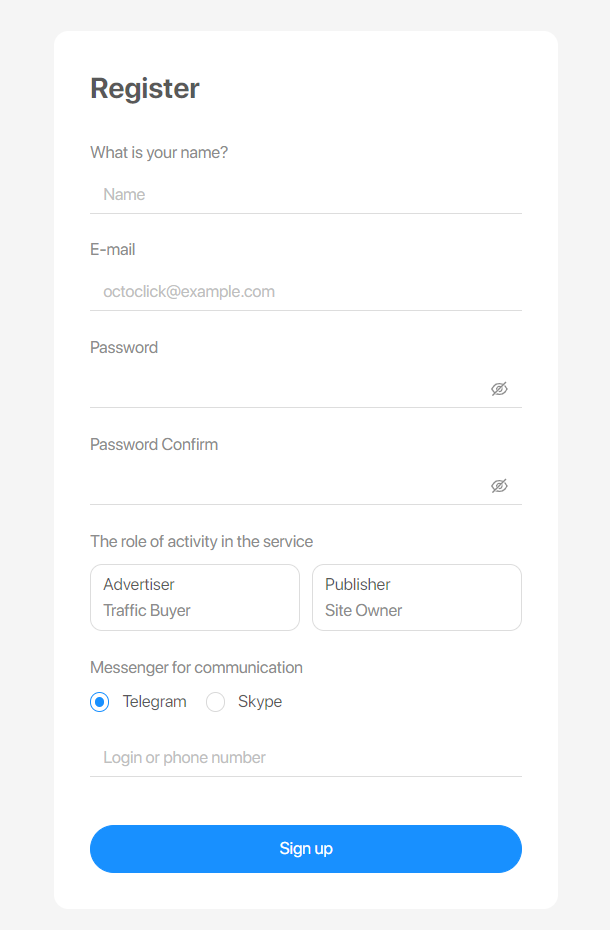This image showcases a registration web page titled "Register" against a clean, white background with varying intensities of gray text. At the top, the page invites users to enter their details to create an account. The first field asks for the user's name, offering separate fields for entering their name and email address. Below this, users are prompted to input and confirm their password, with an option to toggle visibility for both fields, allowing either masked or visible text entry.

The next section requires users to select their role within the service, providing two buttons labeled "Advertiser, Traffic Buyer" and "Publisher, Site Owner." Following this, users must choose their preferred communication platform, with options for Telegram and Skype; the Telegram button is pre-selected. Below this, there is a field where users can enter either their login ID or phone number.

Finally, at the bottom of the page, a prominent blue "Sign Up" button invites users to complete their registration.